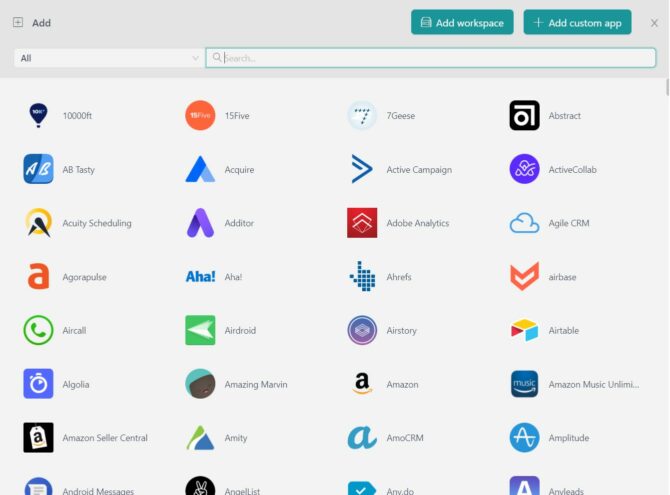The image features a digital interface, likely from a tablet or computer, displaying a variety of app icons arranged in a grid format. The interface design has a light bluish-gray background with a significant banner at the top. In the top left corner of the banner, there are two square buttons labeled “Add” and a plus sign. To the top right, two turquoise buttons are visible, labeled “Add Workspace” and “Add Custom App.” 

Below the banner, a search bar is present with a dropdown option labeled “All” to its left. Underneath the search bar, the main area of the interface is visible, featuring numerous app icons on a light gray background. The icons are organized into four columns and eight rows. Each app icon is accompanied by the app's name. Some of the apps visible in the image include Amazon, Airtable, Aha!, 15Five, Amazon Seller, Aircall, and Abstract, among others.